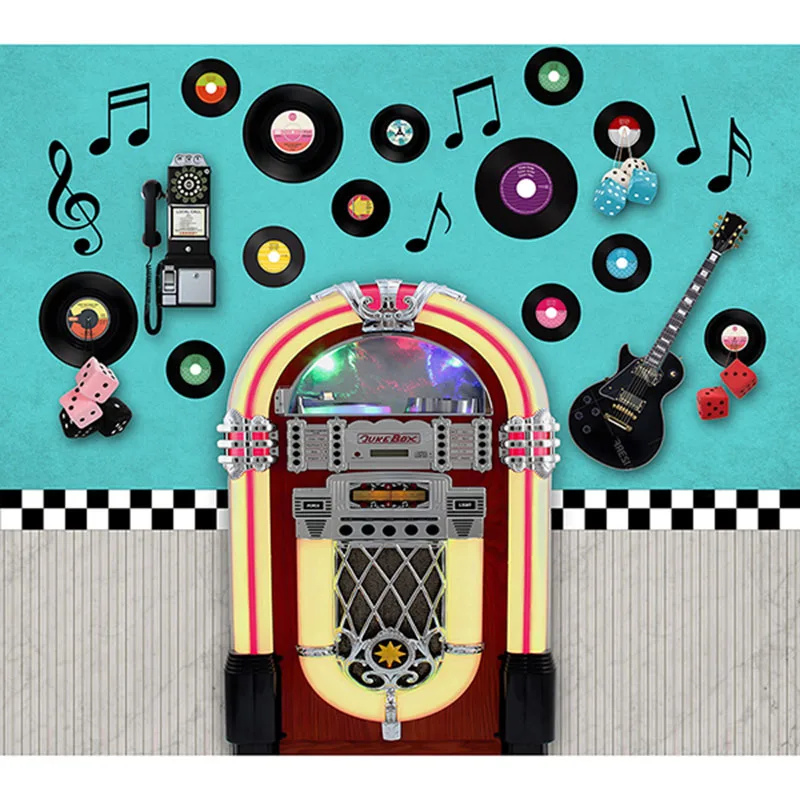This is a detailed photograph of a vintage-style, arch-shaped jukebox centrally positioned in the image. The jukebox features a predominantly redwood-colored body with neon yellow and red arch accents, highlighted with chrome edges and a burgundy face. The center of the jukebox houses a glass section revealing the turntable, while buttons set on a silver plaque allow for song selection. The speaker resides at the base, accompanied by an upside-down U-shaped neon light, and the jukebox stands on black feet.

The wall behind the jukebox is split by a black-and-white checkerboard pattern. Above this pattern, the upper half of the wall is painted a light turquoise, adorned with suspended records of varying sizes, musical notes, a guitar, a pair of red dice, and a rotary payphone. Below the checkerboard line, the wall features vertical gray stripes that run continuously across. The overall artistic style of the image leans towards a stylized, slightly unrealistic depiction, enhanced by the vibrant colors and nostalgic elements that evoke a retro ambiance.